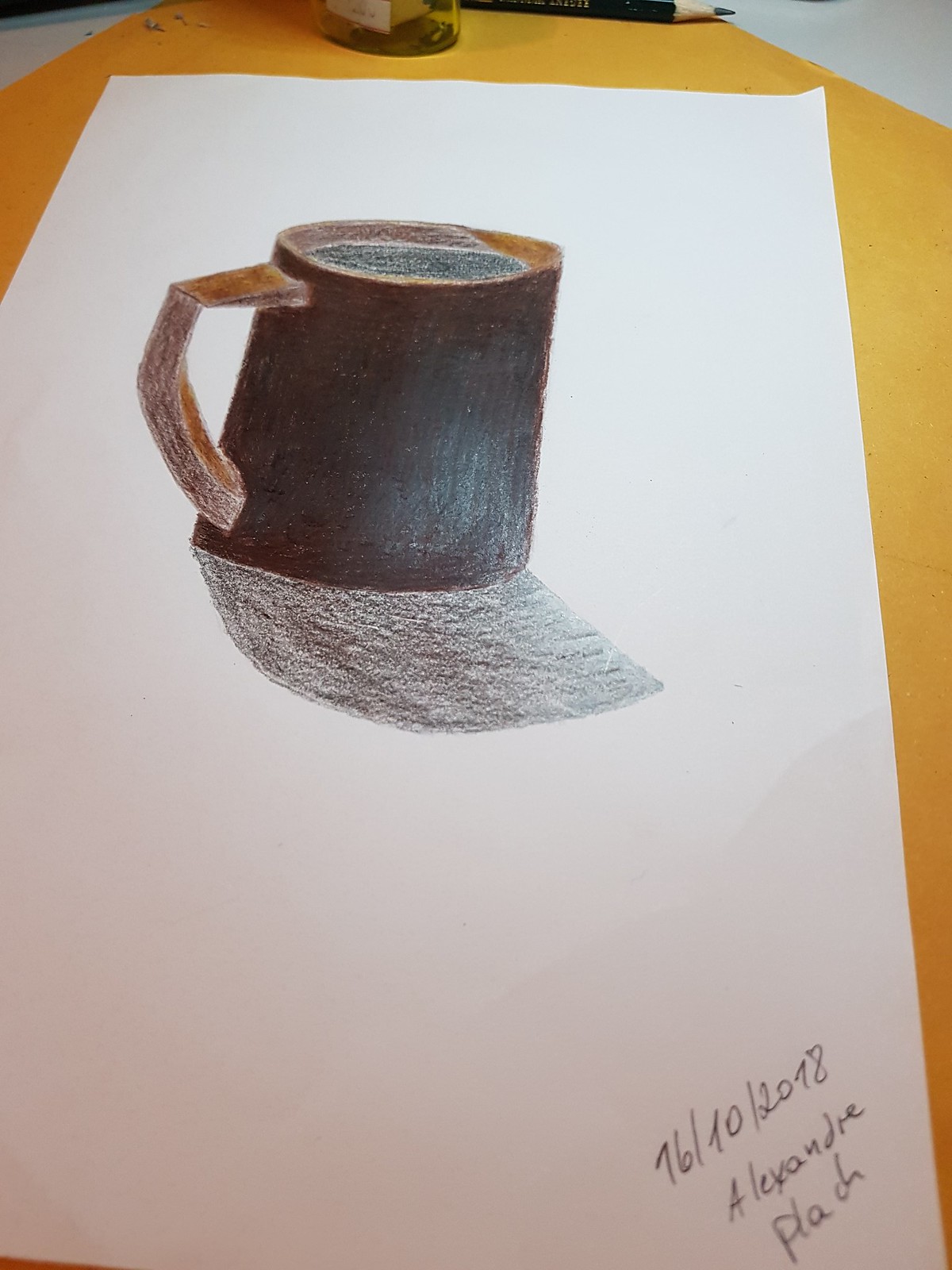In this photograph, an artwork is displayed prominently. The artwork is executed on a large white sheet of paper that is placed over a yellow sheet on a table. At the top of the image, a black colored pencil and a small pencil sharpener rest on the yellow paper. The main focus is a detailed drawing of a coffee mug on the white paper. The mug, rendered in rich dark brown hues, features a handle extending to the left side. The interior of the mug is depicted in a lighter shade of brown, indicating it is filled with coffee. A meticulously drawn shadow extends from the mug, angling downwards and to the right, adding depth to the composition. The artwork is signed "Alexandrae Plock" and dated "October 16th, 2018" in the lower corner.